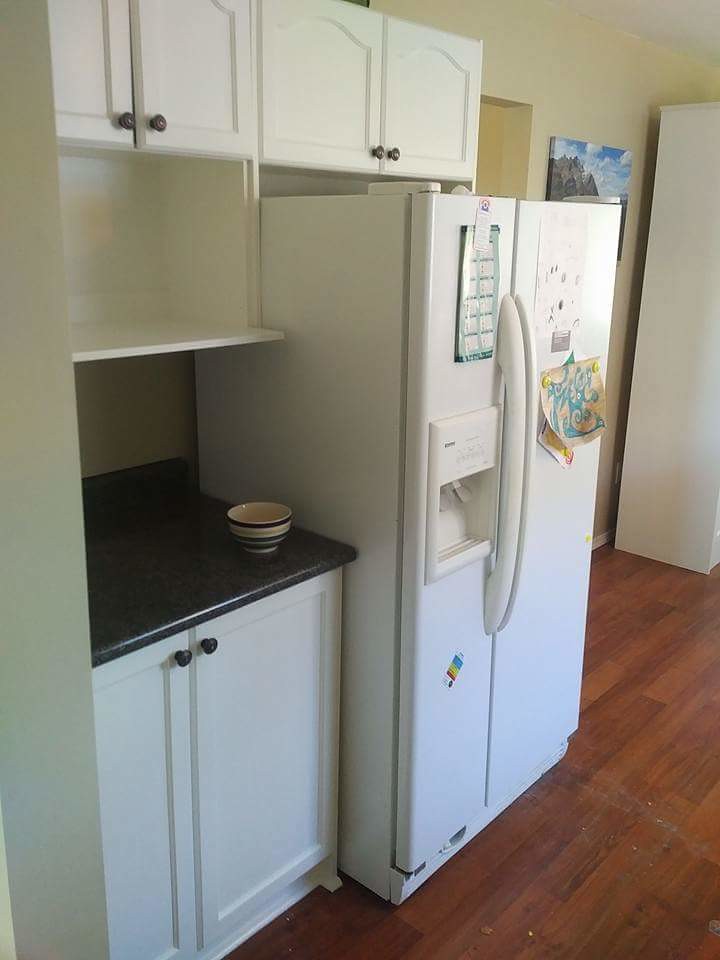The photograph depicts the interior of a kitchen, with a specific focus on the refrigerator area. The refrigerator is a simple, white double-door model equipped with a water and ice dispenser on the left door, featuring long white plastic handles. Adorning the surface of the fridge are several items: a small calendar, a couple of children's drawings, some magnets, and a rainbow-colored sticker. Above the refrigerator, there are white cabinets, and to its left, additional cabinetry follows the same white color scheme with black knobs. These cabinets, positioned above and below, frame a blackish marble countertop. Resting on this counter is an empty, medium-sized ceramic bowl with attractive yellow and blue stripes. The kitchen floor is made of well-worn wooden panels, likely cherry wood. In the background to the right, partially obscured by the refrigerator, is a light yellow wall displaying a landscape painting of sky and mountains. Additionally, an open doorway leads to another room, contributing context to this well-used, cozy kitchen space.